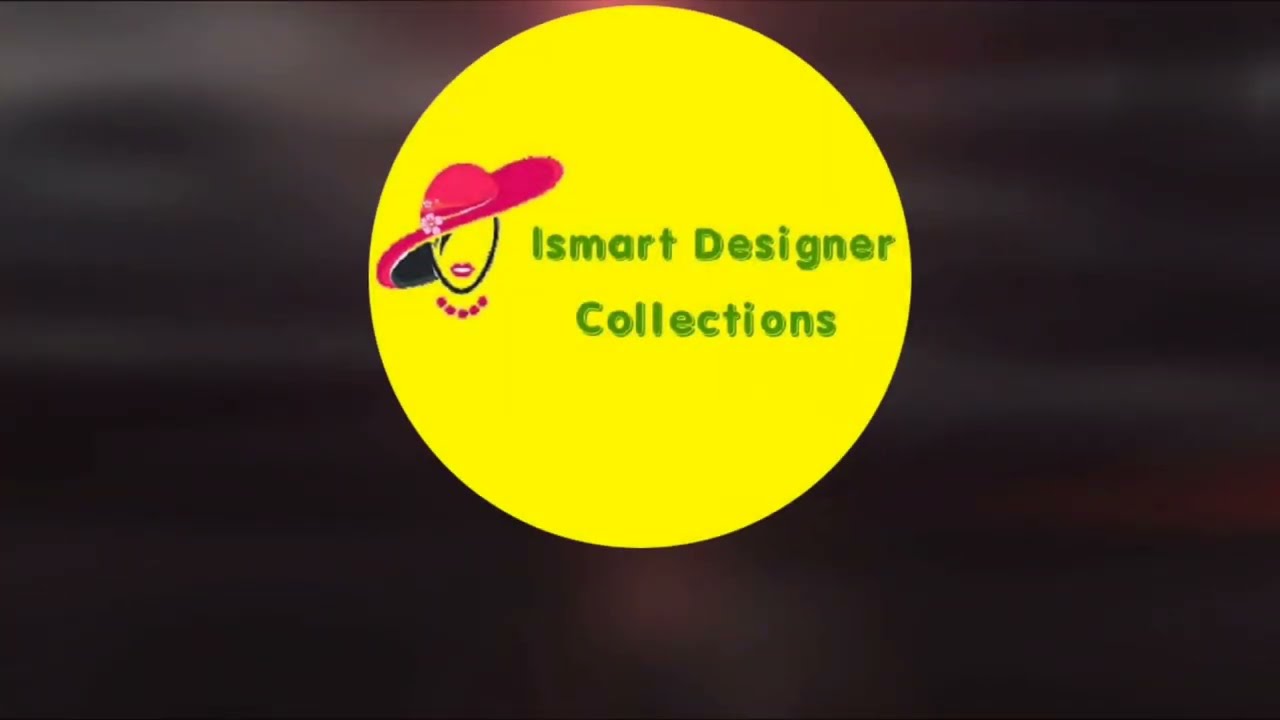The digital image features a dark background with wavy strokes of gray and hints of red. At the center of this backdrop is a solid, bright-yellow circle. Within this circle, there is a digital drawing of a woman's face with a distinctive pink hat adorned with a rose or pink petals, matching hot pink lips, and a pearl necklace composed of pink pearls. Her dark hair, styled with side bangs, partly peeks from underneath the hat. Overlaying the image, in a green, comic-style font, is the text "Ismart Designer Collections." This artwork likely serves as a logo for the mentioned brand.